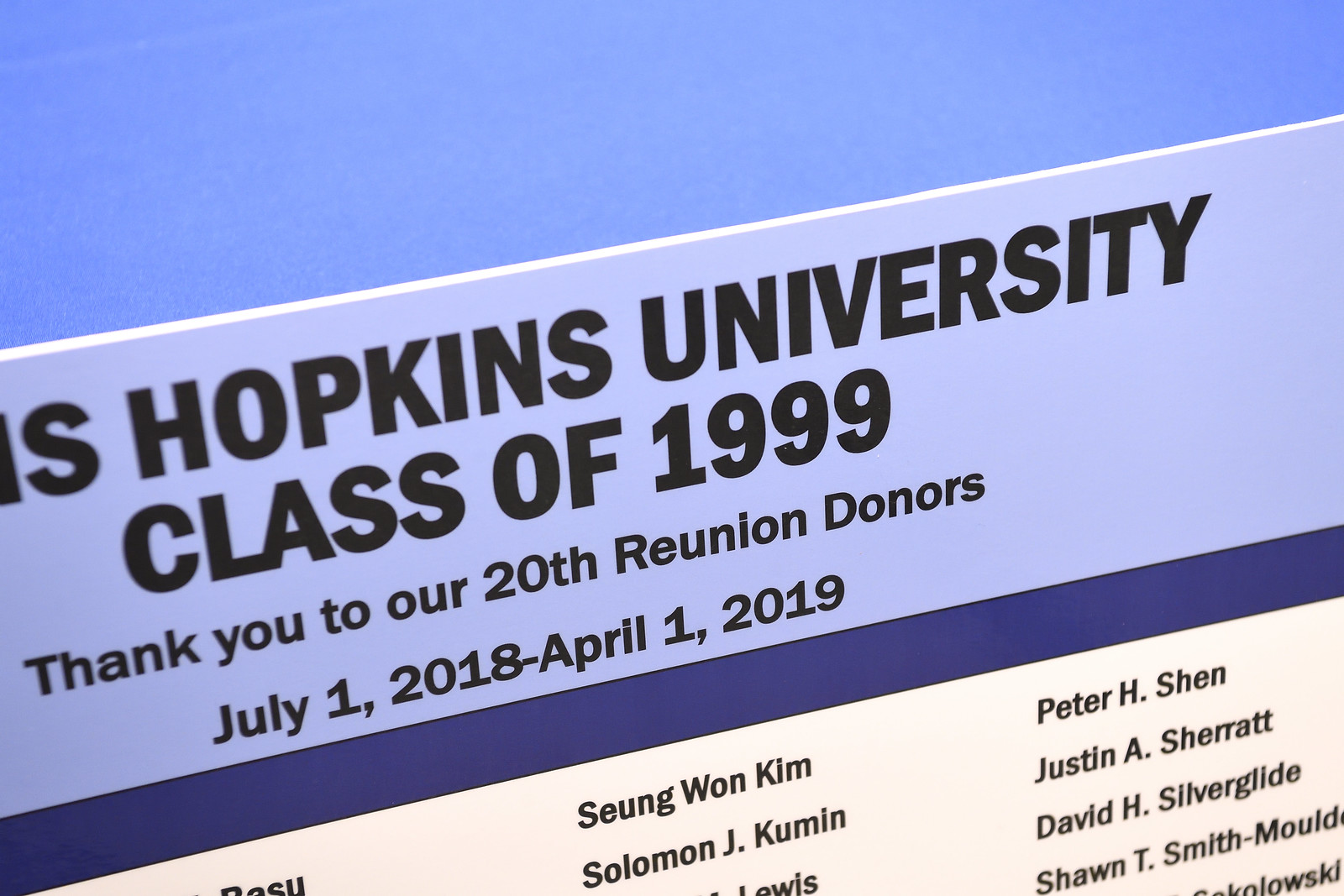The image depicts a sign slanted diagonally from the lower left to the upper right, set against a solid sky blue background. The top section of the sign features the end of some text, prominently displaying the letters "IS" followed by "Hopkins University" in large black letters. Directly underneath, "Class of 1999" is written in bold. Below this, in smaller black letters, it reads "Thank you to our 20th reunion donors" with the timeframe "July 1st, 2018 - April 1st, 2019" following beneath. A thick navy blue line separates this text from a list of donor names, which are displayed on a white background in black letters. Visible names include Sung Won Kim, Solomon J. Kumin, Peter H. Shen, Justin A. Sherat, David H. Silverglie, and Sean T. Smith-Moody. The upper portion of the image also includes a plain blue triangle, serving as a background element. Some donor names are partially cut off due to the angle of the photograph.